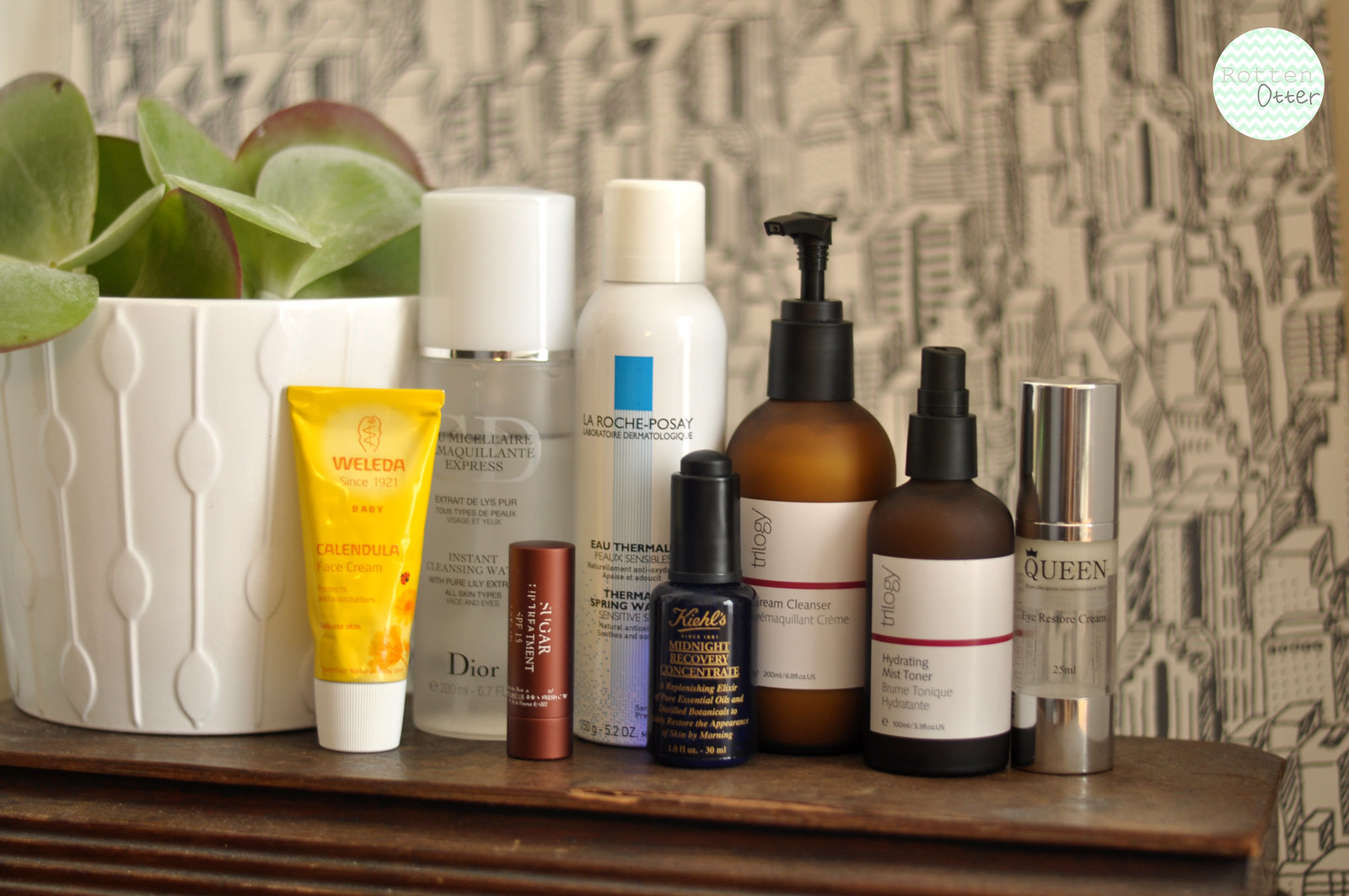On a rustic brown wooden shelf, marked with charming scuffs, sits an eclectic collection of bottles and containers. The backdrop is an elegant gray and white wallpaper, adorned with intricate pencil etchings of variously styled buildings, adding character to the scene. 

At one end of the shelf stands a large white plastic planter with an intricate, repeating design of thin tubes and ovals wrapping around its circumference. From the planter emerges a vibrant green plant, bringing a touch of nature to the curated display.

Next to the planter, several distinct containers are neatly arranged. First, a bright yellow container labeled "WELEDA" catches the eye. Beside it is an elegant see-through bottle from Dior, designed with a white cap and a silver rim, suggesting it might be a spray bottle. An aerosol can bearing the brand "La Roche-Posay" features a sleek, tapered white design.

Adding a touch of earthiness, a small brown container with a black pump is marked with the brand "Trilogy." Next to it is another similar bottle, but in darker glass, also branded "Trilogy." Another aerosol container, labeled "The Queen," stands prominently, conveying a sense of majesty.

In front of the arrangement is a burgundy tube that appears to be a luscious shade of lipstick, and next to it, a diminutive black bottle—possibly nail polish—rounds out the diverse collection. This assembly of containers tells a story of beauty and self-care, set against a backdrop that merges the rustic with the urban.